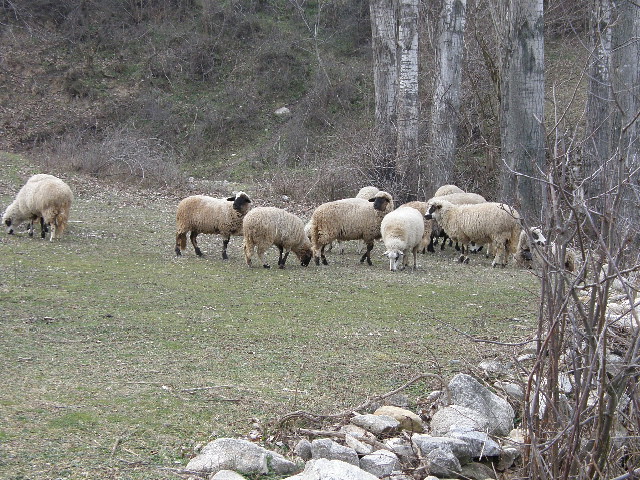The photograph captures an outdoor scene during what appears to be late fall or early winter. The landscape features a mix of faint green grass and patches of brown, indicating dying vegetation. Scattered around the area are big rocks and a hillside dotted with dead bushes and leafless tree trunks that are predominantly gray with hints of white. In the center of the frame stand approximately ten sheep. The majority of these sheep have white bodies with black faces, although there are a few exhibiting a mix of black and white facial patterns or entirely white faces. One distinct sheep with a white face stands apart from the cluster on the right. Most of the sheep are either grazing or lying down, with three of them notably looking in the same direction. Their winter coats are visibly growing in, adding to their fluffy appearance. The scene conveys a serene yet chilly atmosphere, underscored by the bare trees and muted colors.